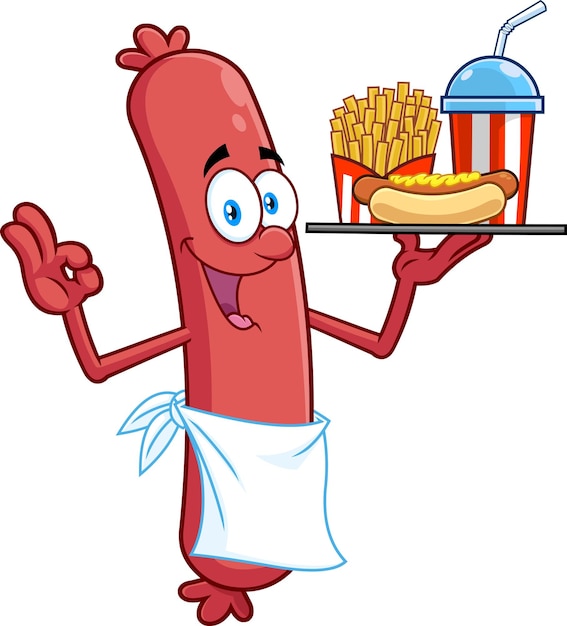This charming animated image features a cartoon hotdog character with a delightful and cheerful demeanor. The hotdog, accented in vibrant red hues, has expressive large white eyes with blue pupils, topped with black eyebrows, and an open, smiling mouth revealing a pink tongue. He is humorously dressed as a waiter, sporting a white apron tied behind his back. 

In one hand, he holds a tray laden with a hotdog adorned with mustard, a serving of yellow French fries in a red and white striped paper carton, and a striped cup with a blue lid and a straw, possibly containing a blue raspberry icy or a milkshake. The paper cup and tray perfectly match his red body with their red and white stripes, creating a cohesive and visually striking appearance. The hotdog's other hand is positioned, making an "OK" sign, adding to his animated charm. The image features no text or background, keeping the focus solely on this endearing, anthropomorphic hotdog waiter.